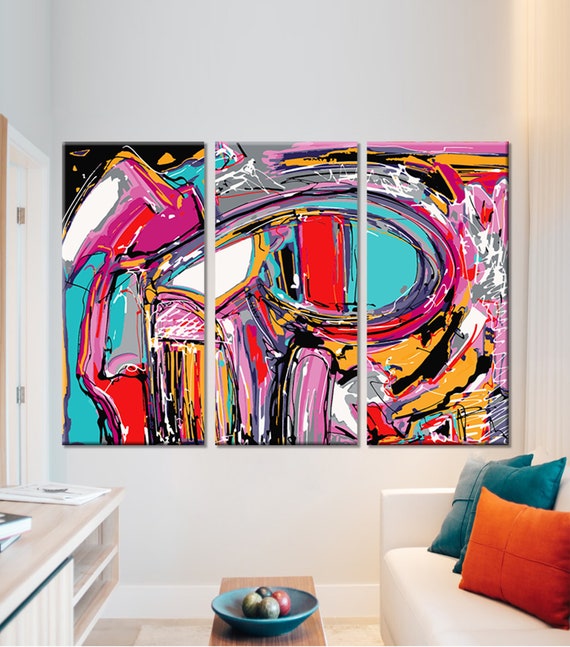The image depicts a cozy, small room that appears to be a family or living room. In the bottom right corner, there's a white sofa adorned with colorful throw pillows in orange, teal, and other hues, though the sofa extends out of the image on the right. Adjacent to the sofa on the left is a small wooden coffee table featuring a green bowl filled with fruit, but this too only partially fits within the frame. To the far left, a white counter with drawers underneath partially appears, and next to it, there's a white door casing leading out of the room.

Dominating the scene is a striking piece of abstract artwork mounted low on the far wall, which is a light gray or ivory color. This artwork consists of three vertical rectangular sections arranged side by side with narrow gaps between them, creating a cohesive and vibrant painting. The left panel bursts with colorful swirls, primarily in teal, pink, red, yellow, and touches of black in the upper corner, reminiscent of graffiti or chaotic energy. The middle panel showcases horizontal bands of color, with red being prominent in the center and darker shades on the extremities. The right panel continues the abstract theme with a dynamic streak of color that arcs downward and then curls back upward at the bottom, dominated by purple, yellow, blue, and red shades.

The room's overall layout suggests a comfortably furnished yet compact space with a blend of practical furniture and expressive decor, exuding a lively and artistic atmosphere.